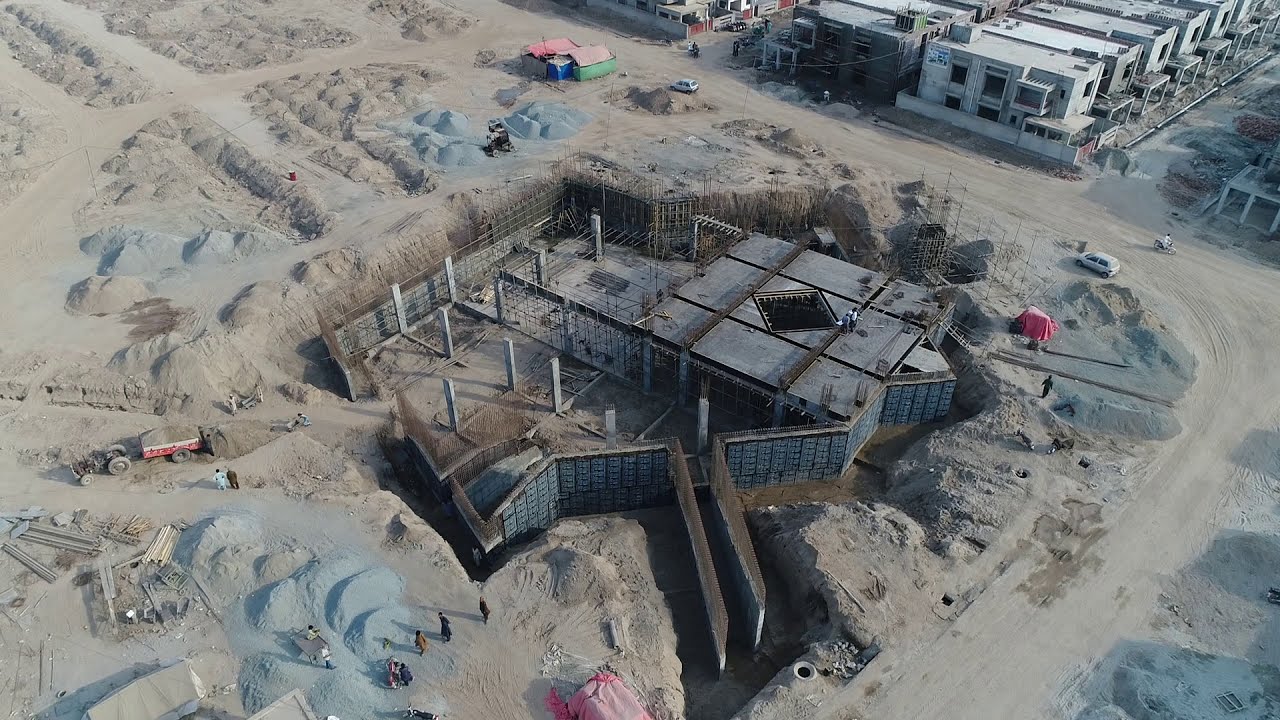The image is a high-angle aerial shot, likely taken from a drone, capturing a bustling construction site situated in the middle of a desert community. The focus is on the foundation work of an expansive building, which features an intricate, almost star-shaped formation with rebar and wood forms outlining its structure. In the center, deep trenches, estimated to be 10 to 12 feet deep, and freshly poured concrete columns suggest the early stages of what will likely be a tall edifice, possibly including an underground garage.

In addition to the central construction zone, the site is surrounded by mounds of cement, sand, and dirt. Various construction vehicles, including haulers, tractors, and trailers, are scattered around, while construction workers congregate near a gravel pile, possibly awaiting deliveries. Adjacent to the main site, rows of completed structures at the top right corner imply a developing residential area. A dirt road encircles the site, with parked cars and additional roadways weaving around the construction zone, giving a sense of a well-organized yet dynamically evolving project.